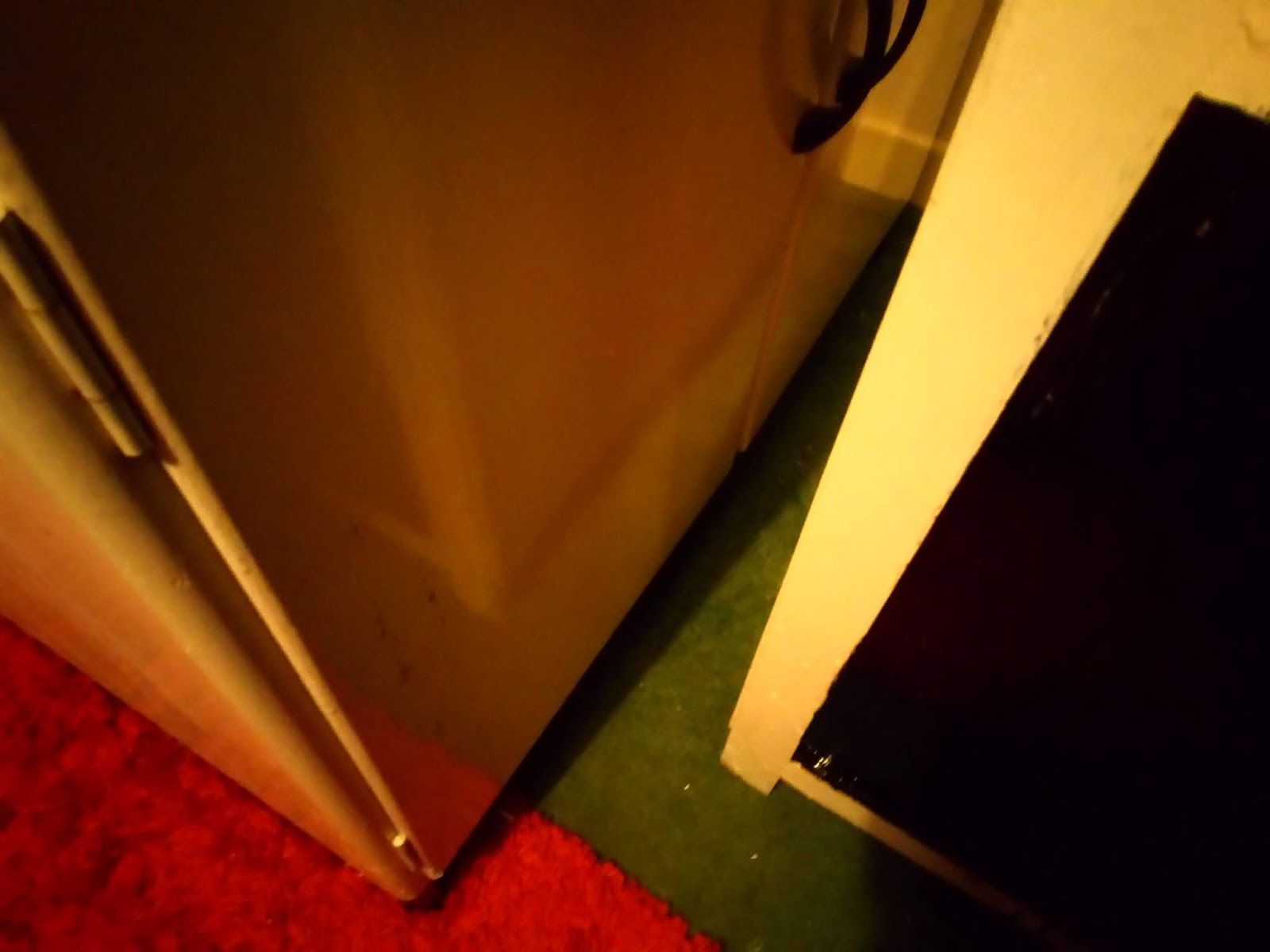The image features an intricately detailed setting with a well-defined foreground and background. In the bottom left and bottom right corners, there are sections of green and red carpets respectively. At the center, a striking cabinet catches the eye; it has gold-colored drawers embellished with black handles on the upper right side. The drawers are adorned with silver hinges along the left edge. 

The cabinet’s reflective surface reveals a secondary yellow cabinet positioned slightly behind it on the left. This yellow cabinet features a draped black cloth cascading down its right side, partially concealing an opening beneath it, as opposed to a standard cabinet door. The yellow cabinet is supported by a small, stubby leg at the bottom. 

In the background, a yellow wall with a yellow baseboard provides a cohesive backdrop. The illumination in the scene creates a shimmering effect on the cabinets, adding depth and visual interest. The gold-colored drawer appears particularly tightly enclosed within the space, indicating it likely cannot be opened.